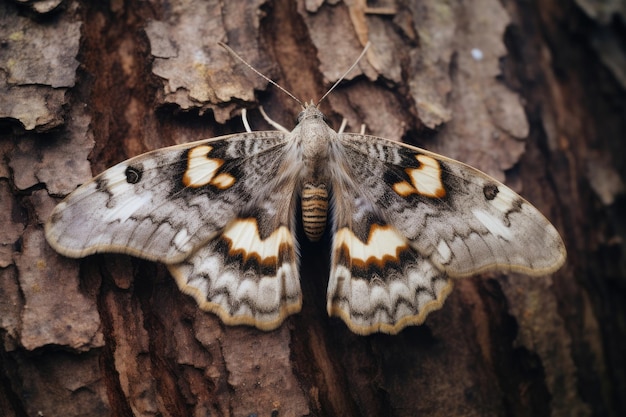This detailed close-up photograph showcases a gypsy moth perched centrally on the textured bark of a tree. The tree bark is a blend of light and dark browns, flecked with patches of peeling bark, which gives an impression of an old and perhaps weathered tree.

The moth is beautifully captured with its wings fully extended, revealing intricate patterns that mimic the bark it rests on. Its wings predominantly feature shades of gray and brown, adorned with delicate wavy and zigzag black stripes, and light tan accents. Notable are the eye-like spots with dark, orange, and reddish markings on the upper wings, adding to its ornate appearance. 

The moth's thorax is striped in hues of yellow and brown, with gray and white fluffy hair. Its body tapers into alternating bands of yellowish-gold, brown, and black, reminiscent of a bee. Two white antennas fan out in a V shape from its head, and its white legs protrude slightly from beneath its body, gripping the bark.

Every detail of the moth, from the gray feathered upper body to the white, creamy, and golden hues on its wings, is meticulously rendered, making it a visually captivating and richly textured image.